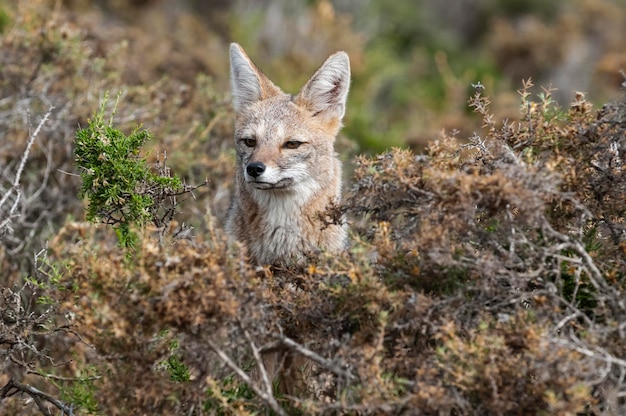In this photo, a young red fox with a mix of reddish, grayish, and whitish fur pokes its head out from the thick brush and foliage of a dense forest. The fox’s face, highlighted by a dark nose and eyes that squint with curiosity, is partially obscured by a tangle of dead brown twigs and brambles. Its small head emerges amidst the brown foliage, drawing attention to the few sprigs of still-green leaves to the left of the frame. The background, filled with more blurred foliage, suggests a deep, wooded environment. The fox appears to be staring slightly off to the left, its ears pricked up and mouth closed, possibly in search of food or simply surveying its surroundings in the midst of this brambly thicket.